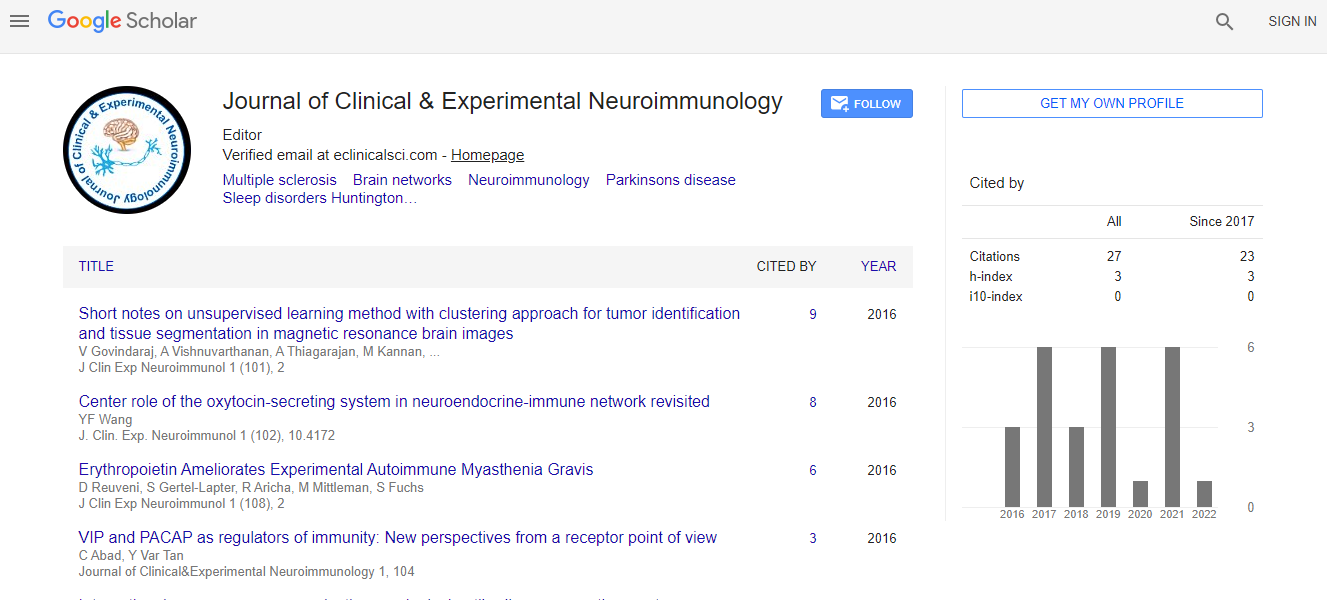Screenshot of Google Scholar Profile - Journal of Clinical and Experimental Neuroimmunology

The image is a detailed screenshot from Google Scholar displayed on a computer screen, showcasing the profile page of the "Journal of Clinical and Experimental Neuroimmunology." 

Located at the top left corner, there's a distinctive white circle with a black outline containing the journal's name. Directly beneath the title, viewers can spot a prominent "Follow" button, and adjacent to it is a large blue rectangular button labeled "Get my own profile."

Further down, the page displays several analytical metrics including citations, H-index, and i10-index. These metrics are visually represented through a bar graph, tracking citation data from 2016 to 2022.

The central section reveals more detailed information about the journal, including an editor-verified email at "clinicalssci.com." The journal focuses on a range of topics such as multiple sclerosis, brain networks, neuroimmunology, Parkinson's disease, sleep disorders, and Huntington's disease.

At the bottom, the page includes four clickable options related to this experimental title, including tabs for "About," "Cited by," and additional insights on the number of citations and the respective years they were cited.